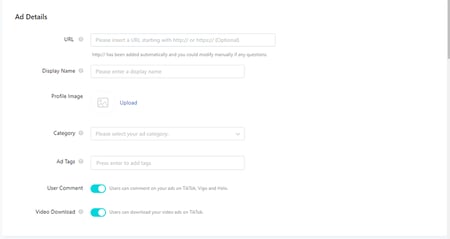The image appears to be a complex layout, possibly a screenshot of a digital interface or form. It features multiple sections and elements with various annotations and symbols. Here is an enhanced and detailed description:

---

The image is a sophisticated digital interface characterized by multiple rectangular sections and lines. Starting from the top, there is a thin gray line running across the left, right, and bottom edges, creating a quasi-rectangular border. Within this border, several areas are highlighted:

1. On the right side, part of this thin line transitions into a thicker gray line, perhaps indicating a section divider.

2. Near the center, a heading or prompt is visible, likely reading "Add details."

3. Below this prompt, there are several segments with structured text. One notable section features a gray-outlined box containing words, followed by another segment of text beneath it. This text is darker, hinting at emphasis or a separate section.

4. Below the emphasized text, there appears to be a circular or dot-like symbol. Nearby, there is another gray-outlined box filled with text, followed by a few more lines of content.

5. Further down, there is distinct text written in blue, suggesting an interactive link or an important note. This is succeeded by another segment of text and yet another gray-outlined box with additional writing.

6. Moving downward, there are more words, followed by a possible symbol, and another gray-outlined box.

7. Towards the bottom right, a blue bar is present, adorned with a white circle outlined in blue. Adjacent to this bar, more text is visible.

8. Below this setup, there is another possible circular or dot-like mark, followed by a second blue bar, also featuring a white circle outlined in blue, with more words to its right.

Overall, the image appears to be an intricate form or user interface, rich in text sections, symbols, and interactive elements, meticulously organized within gray-outlined boxes and blue-highlighted areas.